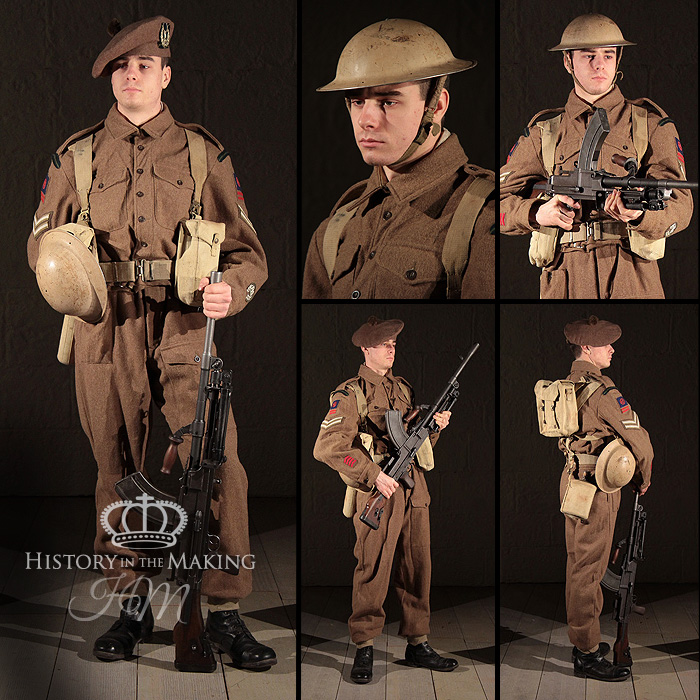In this composite image, five photographs capture a man displaying various military-style outfits and poses, all set against a detailed backdrop. Each photo is marked with a watermark in the bottom left corner, featuring a crown and the phrase "History in the Making HM." The man is consistently attired in a brown uniform, including a buttoned-up shirt with black buttons and matching pants. He pairs this ensemble with black boots and alternates between two headgear: a brown floppy beret and a hard-shell helmet. 

In the full-body shot on the left, the man stands holding a long rifle by the barrel in his right hand while its butt rests on the ground. Straps from his backpack are visible, and the helmet hangs on his left side. The upper torso shot to the right of this displays him wearing the helmet, facing left. Below, in another torso shot, he points the rifle to the right. Meanwhile, the bottom right image shows a side profile of him holding the rifle on the ground with his backpack visible. Finally, the last photo presents him in a diagonal stance, feet slightly apart, gripping the rifle with the barrel pointed skyward. This collection of images, accompanied by the prominent watermark, meticulously showcases the man in different military postures and gear.